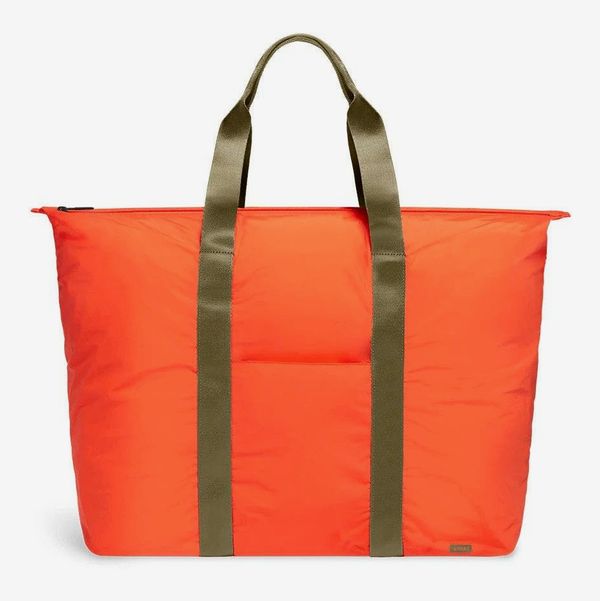The image showcases a large, square tote bag primarily displayed against a plain white background, making it the central focus of the picture. The tote bag is a striking bright orange, crafted from what appears to be insulated, cushioned nylon material, giving it a puffy and squishy appearance. The bag's two brown, almost olive-green straps run parallel to each other and merge at the top to form a singular handle designed for hand-carrying or draping over the wrist rather than the shoulder. The top of the bag features a dark metal zipper, adding to its functional design. Additionally, a small brown name tag label is subtly placed in the bottom right-hand corner of the tote bag. The bag appears simplistic and minimalistic, with visible wrinkles where the fabric folds, enhancing its unpretentious charm. The image is two-dimensional, making it difficult to ascertain whether the bag contains any items.